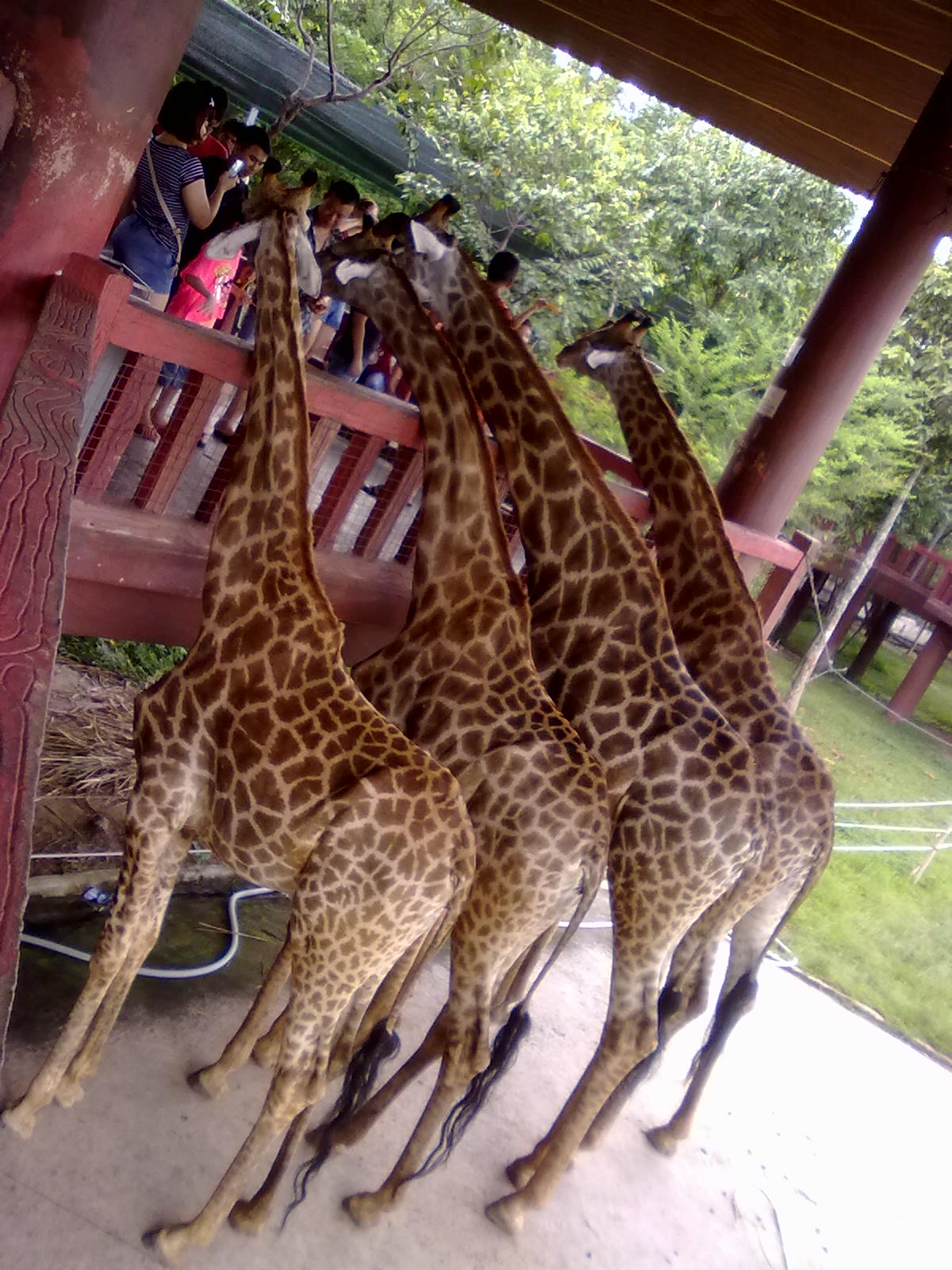In this vibrant and captivating zoo scene, four majestic adult giraffes stand side by side, their long necks extending gracefully over a redwood-colored railing. Their large, curious eyes meet those of the onlooking visitors. The giraffes' distinctive brown and yellow patterned fur glistens in the sunlight, and you can see their black-tipped tails swishing gently. They stand on a beige, concrete floor sectioned off by a white rope fence that runs along the ground. Behind the giraffes, a lush backdrop of trees and grass adds to the naturalistic setting. 

The giraffes are facing a gazebo-like structure elevated on stilts where around a dozen people gather, eagerly snapping photos and seemingly feeding the giraffes. The gazebo, also made of redwood, features a roof that blends seamlessly into the scenic background. Another similar gazebo can be seen in the distance, further enhancing the zoo's enclosed yet open atmosphere. The entire scene exudes an air of tranquility and marvel, capturing a beautiful day shared between humans and these gentle giants.